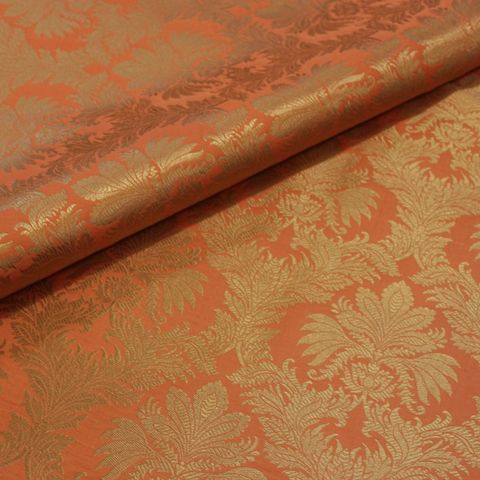The image features a detailed close-up of a floral-patterned fabric, predominantly orange to salmon in color, adorned with light-colored, silvery-gray decorative plants and leaves that cover the entire view. The fabric appears to be a roll extending from the middle of the left side up to the top right corner, bisecting the image with its upward tilt at roughly a 30-degree angle. This roll creates an evident fold or tube-like structure, adding depth and dimension to the scene. The fabric lying flat around the roll seamlessly continues the same intricate floral design, completely filling the frame. The setting suggests a table with the tablecloth unfurled, as the fabric occupies the entirety of the photograph, viewed from a slightly elevated angle, casting subtle shadows on its textured surface.